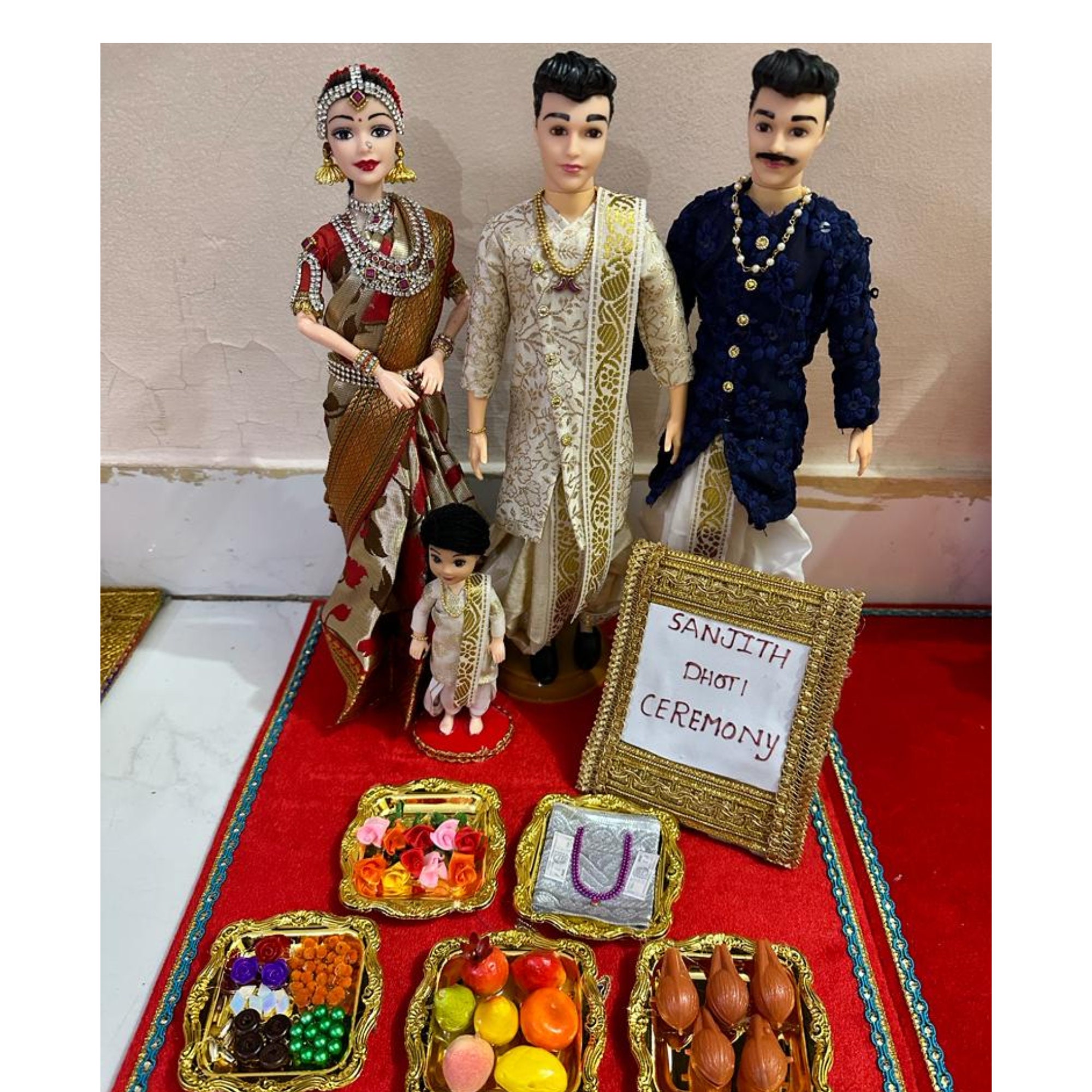The image depicts a detailed scene of four figurine statues set against a beige background, sitting on a red fabric. Three of the figurines are larger and represent adults of Indian or Middle Eastern descent, adorned in traditional Indian attire. The female figure on the left wears a tiara, large earrings, a gown with a wide choker around her neck. The middle figure is a male wearing a white robe, gold necklace, and pendant. The male on the right sports a mustache, a blue robe, and white pants with gold embroidery, accessorized with a distinct necklace. In front of the adults stands a smaller figurine of a child, wearing an outfit similar to the male in the middle. Positioned before them is a golden sign framed with intricate design reading "Sanjith Dhoti Ceremony." Spread in front of the figurines are five golden trays carrying items like colorful flowers, food, and other offerings.